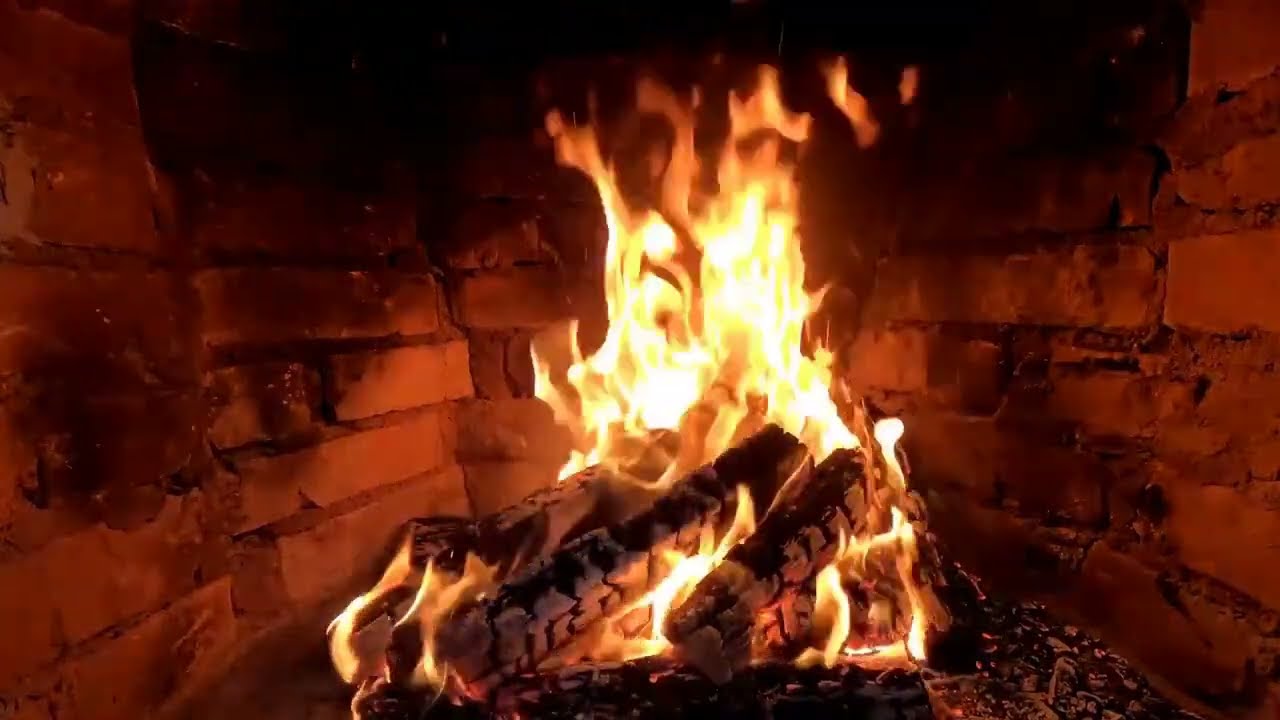This photograph captures an inviting scene of a brick fireplace with a lively fire at its heart. The fireplace is composed of long horizontal reddish-brown bricks, which gain a more vibrant red hue from the fire they contain. Heavily charred logs are artistically stacked at the center, engulfed by bright, licking flames that transition from white and yellow at the base to a slightly more orange hue towards the top. Above the logs, the bricks show signs of blackening from soot and smoke, a testament to many fires past. The base of the fireplace features a half-circle space filled with mulch and smoldering ash, highlighting the intensity of the burning embers. Surrounding the blaze, the bricks curve back on the left before coming forward again on the right, focusing attention on the warm, crackling centerpiece. The image evokes an aura of cozy warmth, typical of a home, with the fire casting a spectrum of colors including deep red, brown, black, gray, a vivid yellow, and the occasional bright white.